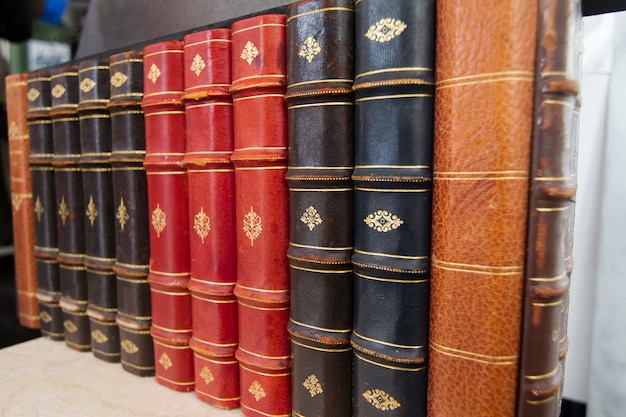This indoor photo, taken at a slightly angled perspective from the right, showcases a set of antique-style leather-bound books neatly arranged on a beige-colored bookshelf or table. The collection appears to be well-preserved, suggesting they are quite old, possibly dating back to the 1800s. The books are arranged in a specific order: starting from the left, there's a brown (or gold) book, followed by four black books with golden accents, then three red books with similar gold detailing, proceeded by two more black books, and concluding with another brown (or gold) book. They stand upright, their consistent and ornate logos indicating they may be part of a complete set, though possibly from different sub-series within the collection. In the upper left corner of the image, the darkened background hints at additional books, suggesting the scene might be a library.